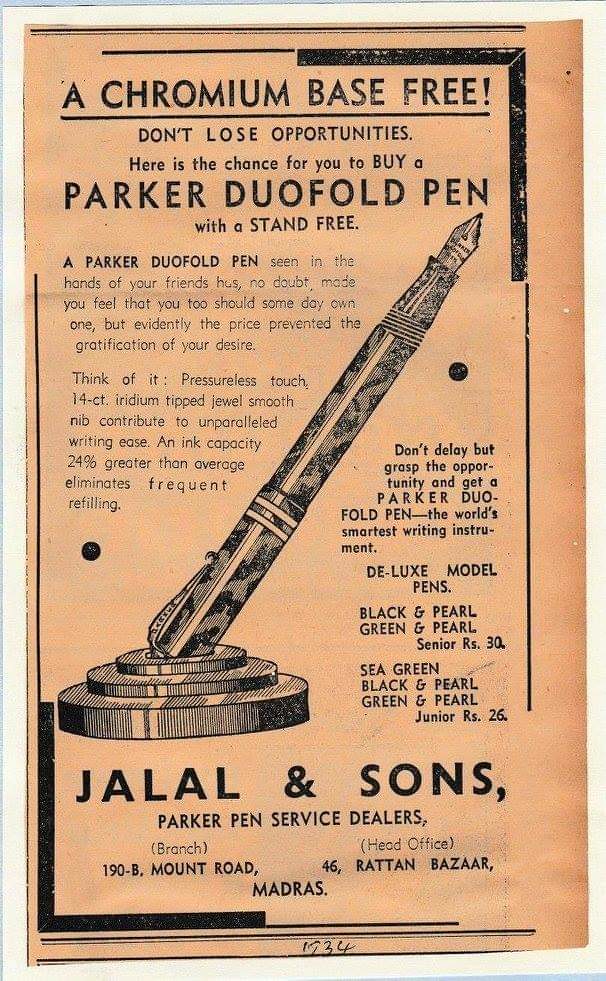The image is an advertisement or flyer for a Parker Duofold pen displayed on a faded orange or peach-colored background. The flyer features bold black text at the top declaring "Chromium Base Free. Don't Lose Opportunities." It encourages potential customers with the message, "Here's the chance for you to buy a Parker Duofold pen with stand free."

Below this text, there's a detailed black-and-white illustration of the pen prominently displayed in its stand. The pen is described as "the world's smartest writing instrument" with unique features including a pressureless touch and a 14-carat iridium-tipped jewel smooth nib offering unparalleled writing ease.

Further down, the flyer identifies the seller as "Jalal and Sons Parker Pen Service Dealers," providing both their branch and head office addresses in Madrid, Spain. The advertisement also emphasizes not to delay in purchasing, stating "Don't delay, but grasp the opportunity and get a Parker Duofold pen." The pen is available in various luxurious styles such as black and pearl, green and pearl, sea green, black and metal, and green pearl. The advertisement dates back to either 1917 or 1934, as indicated at the bottom of the flyer.